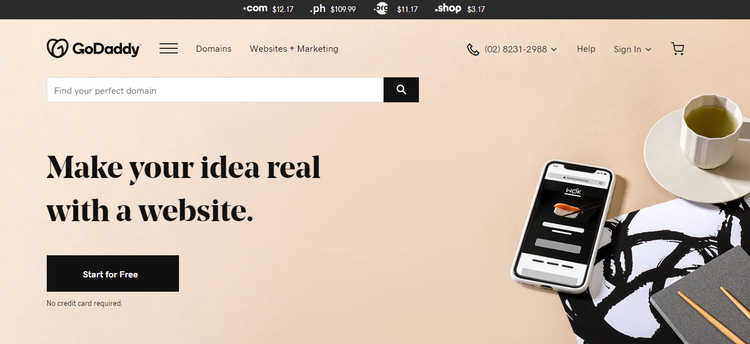This screen capture displays the GoDaddy website, characterized by its beige background with a dark gray header and black text. The webpage features a combination of images situated primarily in the lower-right and upper sections. 

In the lower right, a stylized, Photoshopped image presents a placemat, white with black swirling paint stripes. Atop the placemat rests a neatly folded gray napkin, which supports two tan-colored, wooden chopsticks laid across it. Hovering over the upper right corner of this setup is a teacup—a round, white cup with vertical ribs, filled with a greenish tea, and placed on a matching round saucer. 

An additional visual in the upper left shows a cell phone screen displaying a website featuring an image of sushi. This complements the desktop view wherein the prominent GoDaddy header includes a search bar situated on the upper left. Below the bar is a motivating tagline in bold black text that reads, "Make Your Idea Real with a Website," followed by a bold black button with white text stating, "Start for Free."

The screen capture, roughly twice as wide as it is tall, encapsulates GoDaddy's blend of functionality and inspirational imagery, aimed at encouraging viewers to bring their creative ideas to life through an online presence.